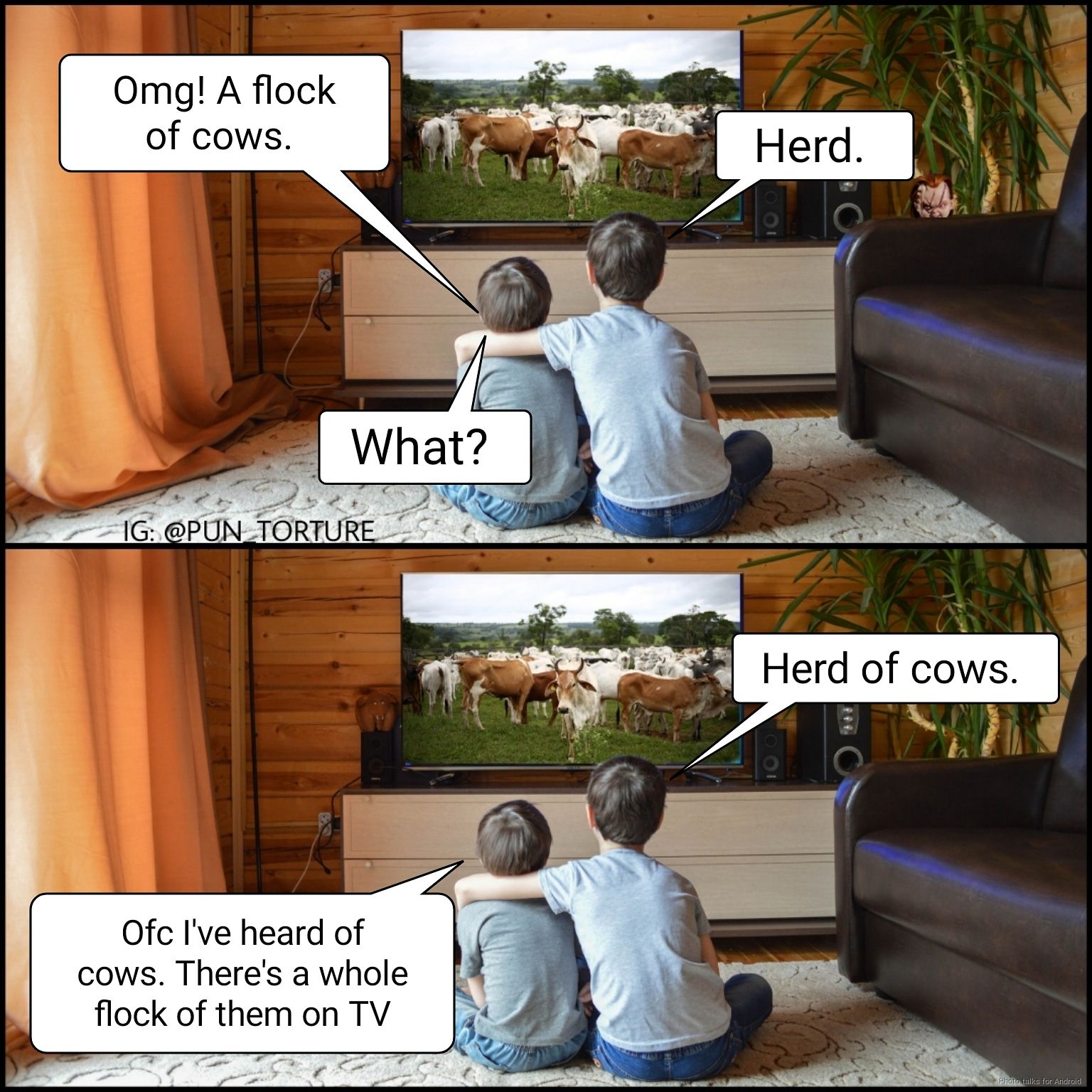The image is a meme with two identical segments, one above the other. Both segments feature two young boys, approximately aged five and eight, sitting on a white rug in a living room, watching TV. The boy on the left is in a light blue shirt and jeans, while the boy on the right, who is slightly larger with his arm around the younger boy, is wearing a dark gray shirt.

In the background, there's a black leather chair on the right, a plant, and an orange curtain to the left against a wooden wall. The TV screen displays images of white and brown cattle.

In the top segment, a conversation bubble from the boy on the left exclaims, "OMG, a flock of cows." The boy on the right corrects him with, "Heard." Confused, the boy on the left responds, "What?" The boy on the right clarifies, "Herd of cows."

In the bottom segment, the boy on the left says, "OFC, I've heard of cows. There's a whole flock of them on TV." To which the boy on the right reiterates, "Heard of cows." The meme humorously plays on the pun between "heard" and "herd."